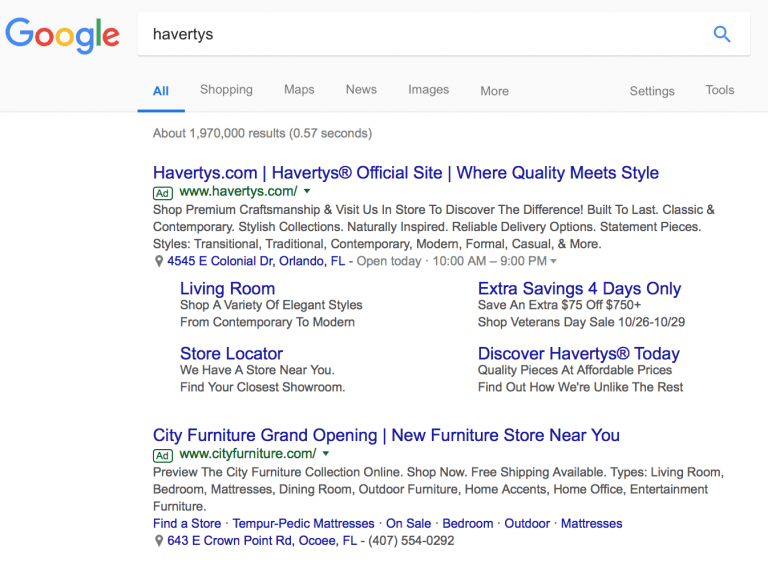The image is a rectangular screenshot of a Google search results page, likely captured from a web browser such as Chrome. The layout follows the conventional Google interface with a light gray border running horizontally across the top. On the top left corner, the recognizable "Google" logo is prominently displayed. Adjacent to the logo is the search query box containing the keyword "Haberties," complemented by a blue search icon on its right.

Below the search bar, there is a navigation menu with categories including "All," "Shopping," "Maps," "News," "Images," "More," "Settings," and "Tools." The "All" category stands out in blue with an underline, indicating it is the currently selected option.

The search results display approximately 1,970,000 results generated in 0.57 seconds. The first result features a promoted link titled "Haberties.com, official site - where quality meets style," marked with an "Ad" label and the URL "www.haberties.com." The second result advertises "City Furniture Grand Opening," describing a new furniture store near the user's location.